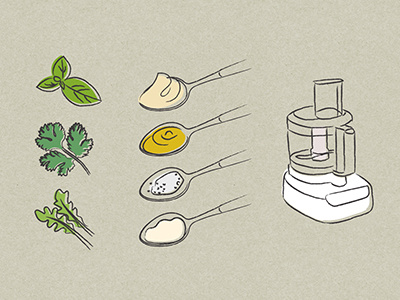This illustration features a detailed arrangement set against a gray background, showcasing three different herbs and a food processor. To the left, three herbs are depicted, possibly mint with its teardrop-shaped leaves, cilantro characterized by jagged edges and small leaflets, and arugula with its evenly spaced, wavy leaves. To the right of the herbs, four spoons are illustrated diagonally from top right to bottom left, each containing a distinct substance. The top spoon holds a creamy substance, likely mayonnaise, followed by a yellow substance that appears to be mustard. The third spoon contains a coarse, spotty white powder that might be sugar or salt, and the bottom spoon also has a creamy or mayonnaise-like substance. To the far right, a food processor is illustrated with a white base, a clear top, and a white center with visible blades, contrasting with the gray background.